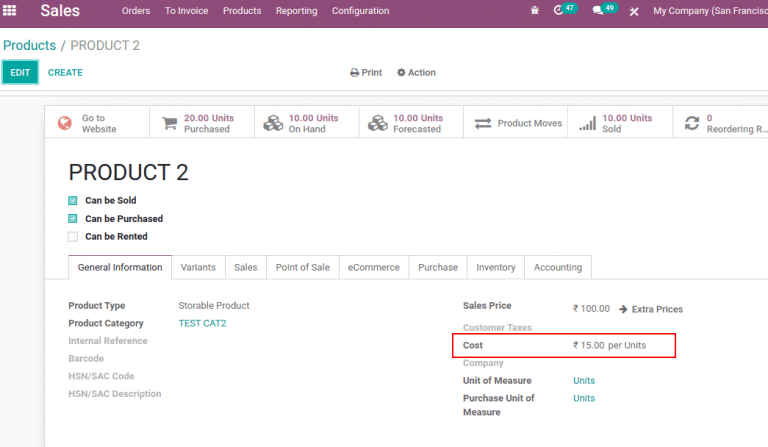The image showcases a product sales page from a company based in San Francisco. At the top of the page, there is a prominent purple bar featuring various headings. On the right side of this bar, the company name "My Company San Francisco" is displayed. The product listing falls under the category "Products," which is highlighted in turquoise.

The focus is on "Product 2," which is available for both sale and purchase, though these options have been selected while the rental option has not. Detailed information about the product is provided below, including its classification as a "Storable Product" and its category, "Test Cat 2." The sales price is listed as 100 units of an unspecified currency represented by a unique squiggle symbol. There is an option to reveal additional pricing details by clicking on an arrow.

Additionally, customer taxes are specified, marked in red with the word "Cost," which amounts to 15 units of the same unidentified currency per item. The lower section of the page contains further information, although it is not immediately comprehensible from the description provided.